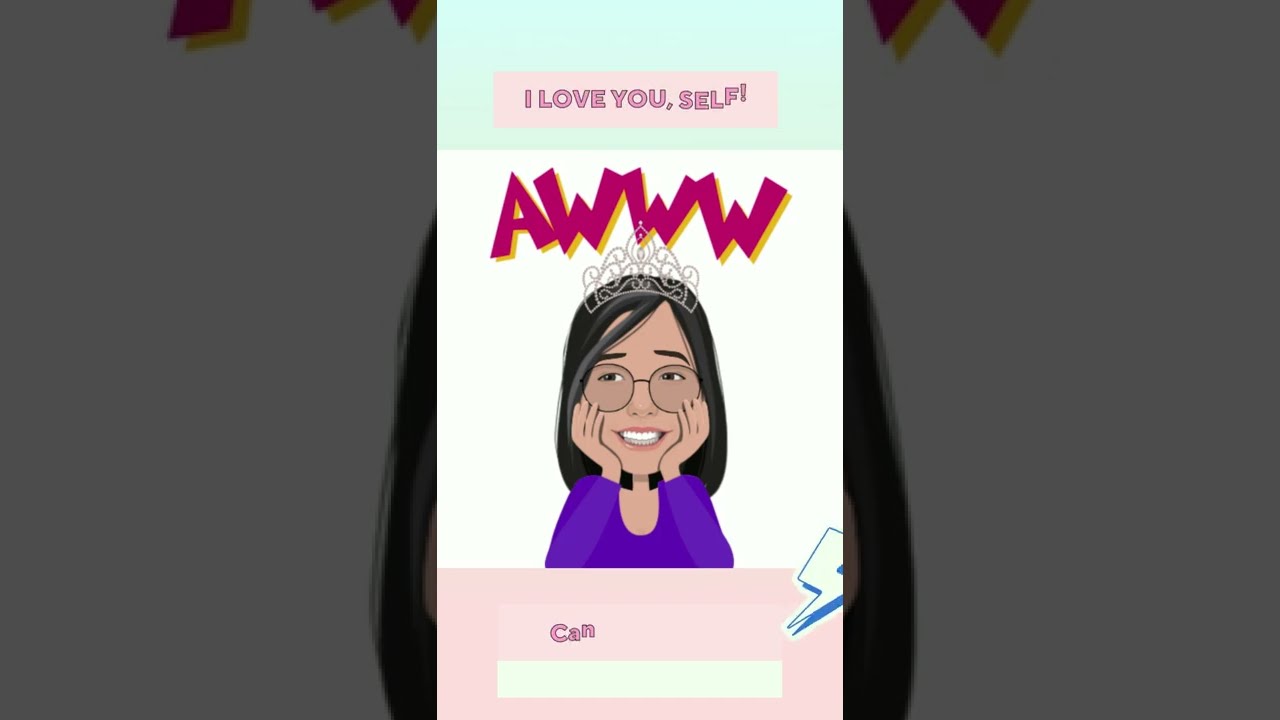The image is a vibrant, cartoon-style digital art piece, likely a screenshot from a smartphone app promoting self-love and positive reinforcement. Dominating the top part of the image, a pink text box with the words "I love you, self" exclamates in white font. Just below this, the phrase "AWWW" is boldly presented in magenta, three-dimensional comic book-style font with a golden drop shadow, set against a white background.

Central to the image is a digital depiction of a young girl with dark black hair and brown skin. Adorned with an elegant silver tiara, she wears round glasses and a black choker necklace. Her hands cradle her cheeks as she smiles warmly. She is dressed in a long-sleeved purple shirt, and her pose projects a sense of comfort and charm.

A secondary text element at the bottom of the image spells out "CAN" in pink letters, accompanied by a white and blue lightning bolt symbol, suggesting empowerment. The entire image is set against a light blue background, with an enlarged, darker version of the girl's face faintly visible in the backdrop, adding depth to the piece.

Overall, the composition combines lively colors and expressive typography to create an uplifting and visually engaging message of self-affirmation.